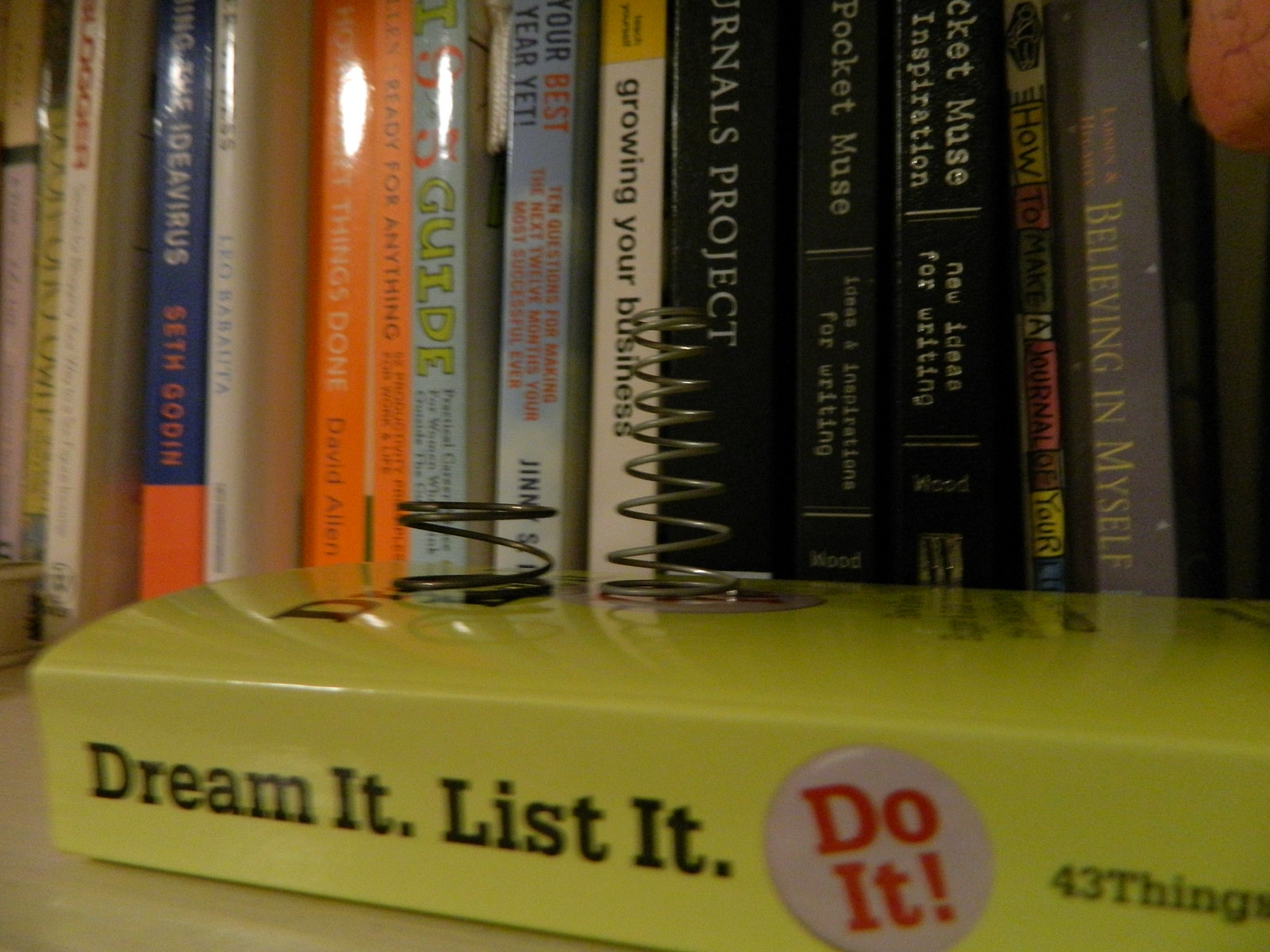In the foreground of this photo, a yellow book titled "Dream It, List It, Do It: 43 Things..." lies flat on its back, displaying both its cover and spine amidst a collection of upright books on a bookshelf. Resting atop this book are two metal springs: the left one is shorter and broader with a dark bronze hue, while the right one is taller, tapering from a wider base to a narrower top in a silver color. The background reveals approximately 15 books, many oriented towards self-help and personal improvement, with visible titles including "Our Best Year Yet," "Growing Your Business," and "Believing in Myself." A few other book titles are partially obscured or have white reflections on their covers, making them difficult to read. The juxtaposition of the springs on the self-help book and the neatly arranged titles behind it creates an intriguing and somewhat peculiar scene.